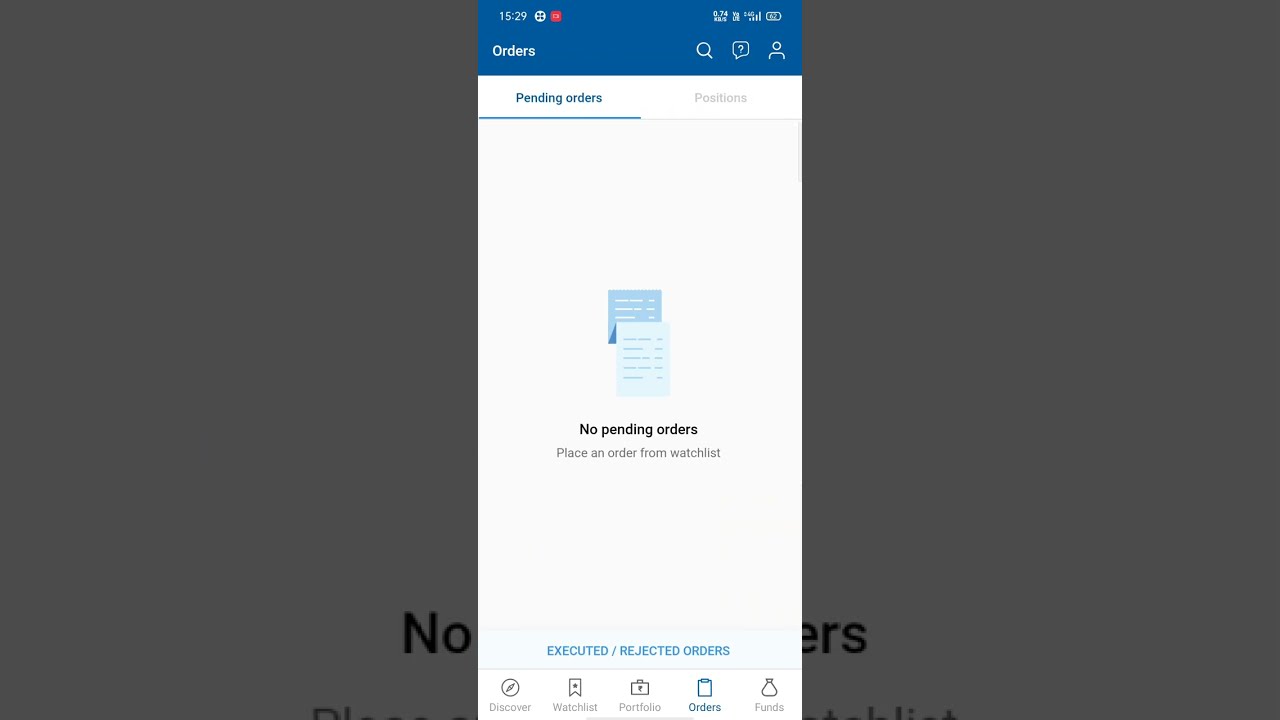The image features a central screenshot of a financial app against a wider, steel gray background with a wide aspect ratio. The top of the screenshot displays a blue header with white text reading "15:29 Orders," indicating the time as 3:20 PM. The battery life is shown at 62%, and all signal bars are present. Icons for a magnifying glass (search), a question mark (help), a speech bubble (messages), and a user profile are aligned at the top right.

The app's main interface has a white background and two highlighted tabs at the top: "Pending Orders" in blue, which is currently selected, and "Positions" in gray. Below this, a central graphical element depicts a folded sheet of paper in shades of blue—a darker blue at the top transitioning to a lighter blue at the bottom. This graphic is accompanied by the text "No Pending Orders, Place an Order from Watchlist."

Further down, blue text reads "Executed / Rejected Orders." At the bottom of the screen, the navigation bar includes five buttons labeled "Discover," "Watchlist," "Portfolio," "Orders," and "Funds." The adjacent wide background only partially displays the words "no" on the left and "ERS" on the right side.